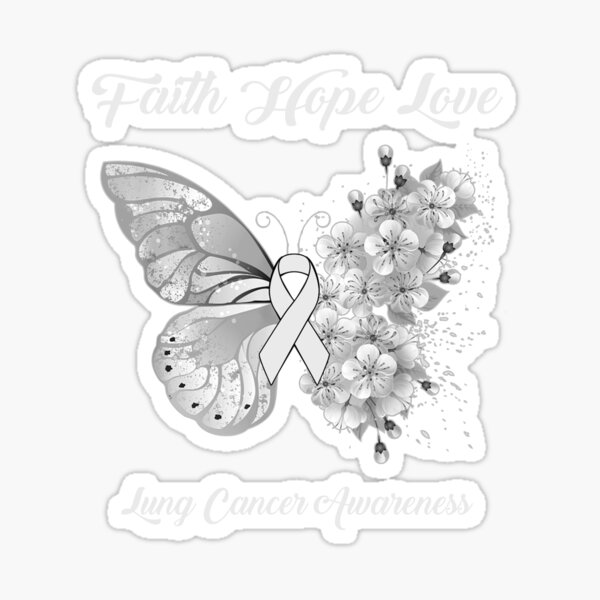The image is a large square graphic with a solid light gray background and no border. At the top, the words "faith, hope, love" are written in gray cursive within a decorative darker gray border against a white background. Below the text, centered in the middle, is an intricate illustration where the left side features realistic-looking butterfly wings with patterns on the upper and lower sections. Connecting the two wings in the middle is a ribbon, representing cancer awareness. Extending to the right side, the butterfly wings transition into a cluster of detailed flowers, shaded in various tones of gray. At the bottom of the image, the phrase "lung cancer awareness" is also written in gray cursive, framed similarly with a darker gray decorative border against a white background. The entire butterfly, including its curled antennae, and the flowers, are shaded solely in light and dark gray, creating a monochromatic effect. The composition visually represents the blending of hope and awareness through symbolic elements unified in a single, cohesive design.